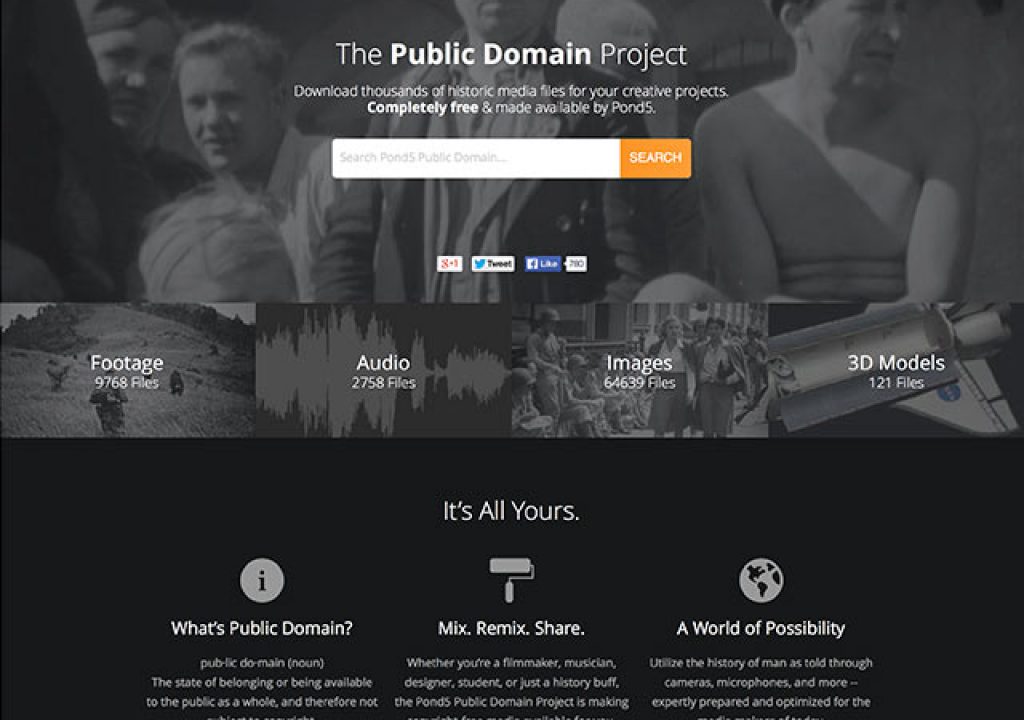This screenshot showcases the Public Domain Project by Pond5. The background features a collage of historic images of various people. Prominently displayed are four main categories—Footage, Audio, Images, and 3D Models—with the tagline “It’s All Yours” beneath them.

An informative graphic explains the concept of the public domain, emphasizing the free and unrestricted use of these resources for creative projects. To the right, it highlights options to "Mix, Remix, and Share," and invites users to explore a "World of Possibility" by downloading thousands of historic media files.

These resources are provided completely free of charge by Pond5, and the platform includes a search bar with an orange search button for easy navigation. The website predominantly utilizes a black and gray color scheme, and includes social media icons for Google, Twitter, and Facebook, allowing users to share their findings.

The database boasts an impressive collection:
- Footage: 9,768 files
- Audio: 2,758 files
- Images: 64,693 files
- 3D Models: 121 files